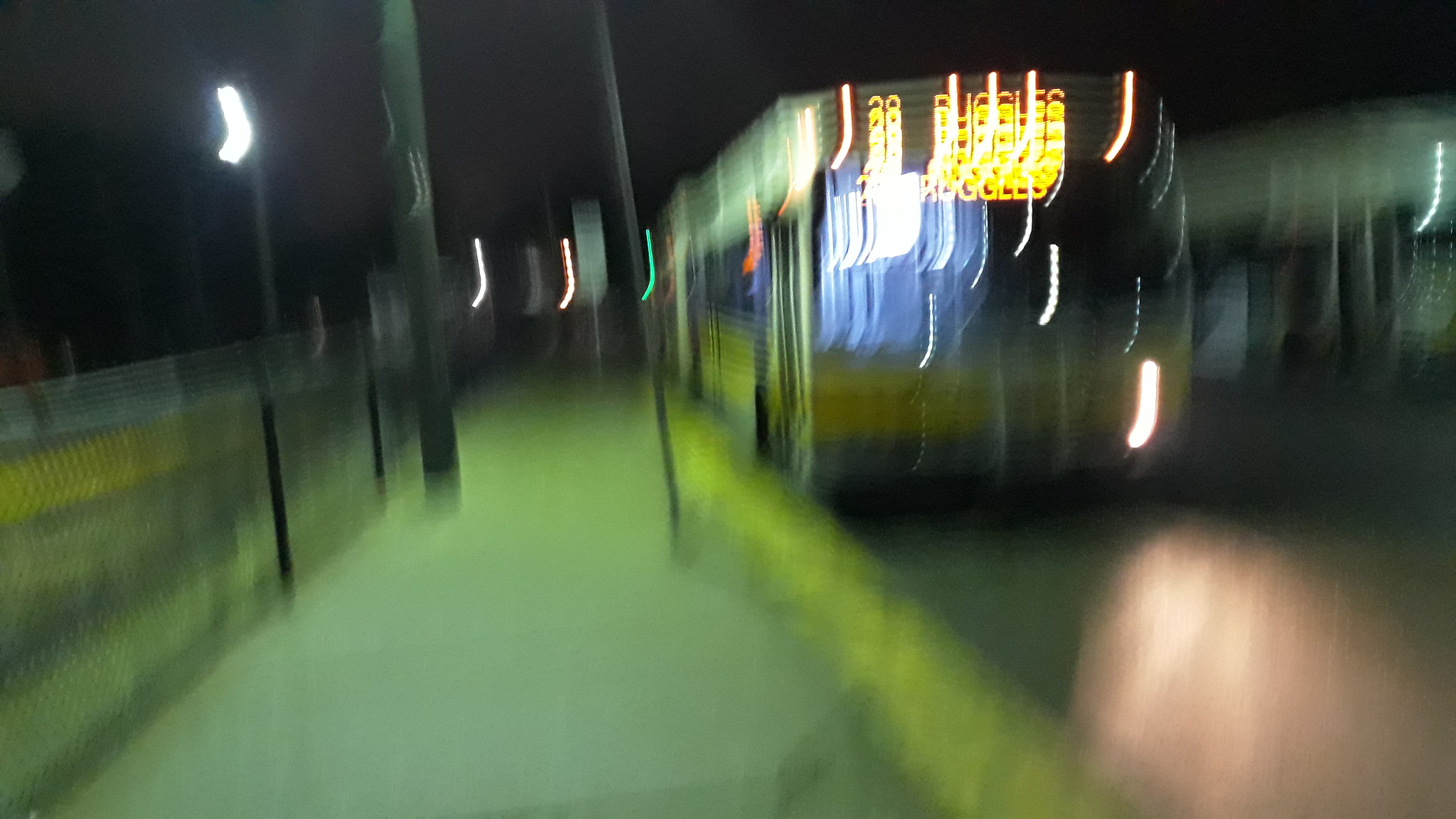This horizontally-oriented, rectangular image captures a low-resolution, extremely blurry photograph of a nighttime urban scene, possibly a side street. The right side of the image features a sidewalk delineated in yellow and flanked by a series of black, narrow streetlights emitting a vertical yellow glow. Adjacent to the sidewalk, a one-story storefront building is faintly visible, adorned with blurred neon signs in yellow, white, and light blue hues. On the left side of the image, what appears to be a fence post can be partially identified. The lower right corner of the image contains a flesh-colored, oblong shape, likely the fingertip of the person who took the photo, adding an inadvertent and personal touch to the scene.